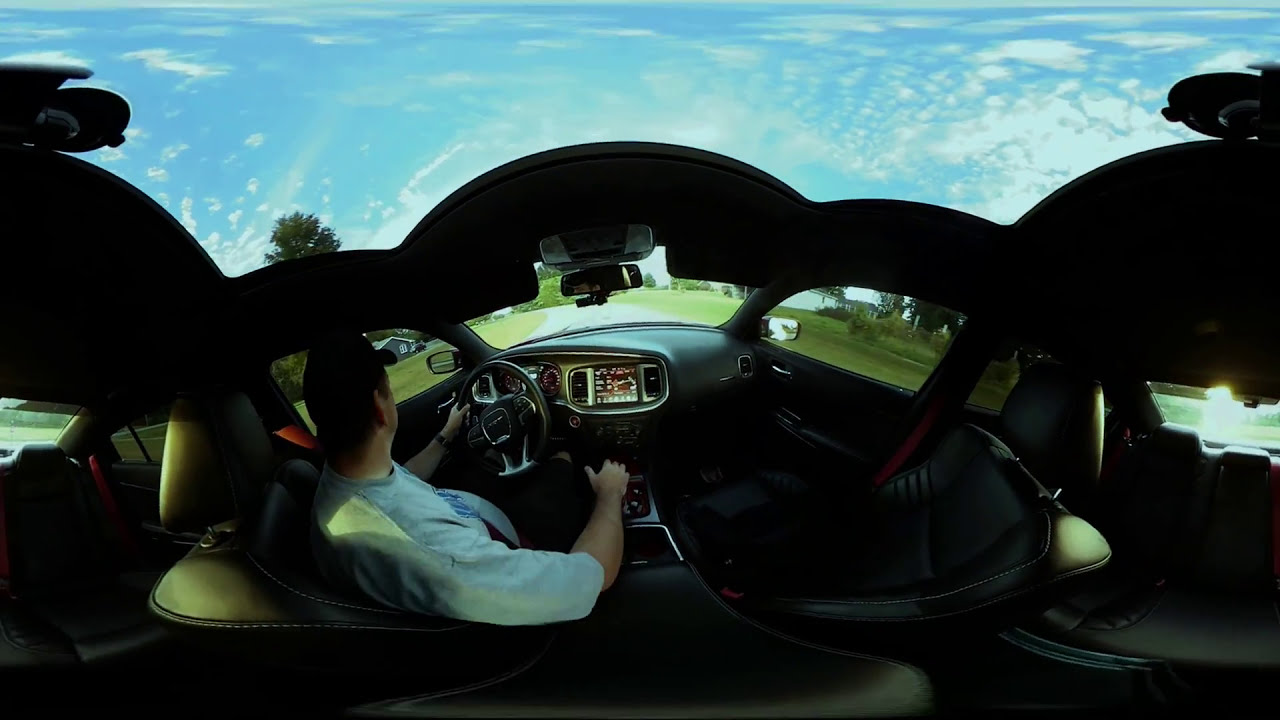This panoramic image, taken from the perspective of the back seat of a car, showcases a detailed and immersive view of its interior and the surrounding landscape. The car's curved shape is accentuated by a lens that widens the foreground, creating a tubular effect. The interior is furnished with black leather seats and a black dashboard. A man is seated in the front driver's seat, wearing a black baseball cap and a gray t-shirt with unreadable text. His right arm rests on the armrest while his left hand grips the steering wheel. A screen with various lit-up text is visible to the right of the wheel.

The top of the car is fully open, revealing a bright blue sky with scattered white clouds which fills the top third of the image. Beyond the windshield, the scenic view includes green grass, tall trees, and houses, with what looks like a driveway stretching ahead. The man appears to be looking towards his left side mirror. The clarity of the image enhances the vibrant colors and finer details, from the greenery outside to the intricate interior of the car. No other people are present in this strikingly clear photograph.